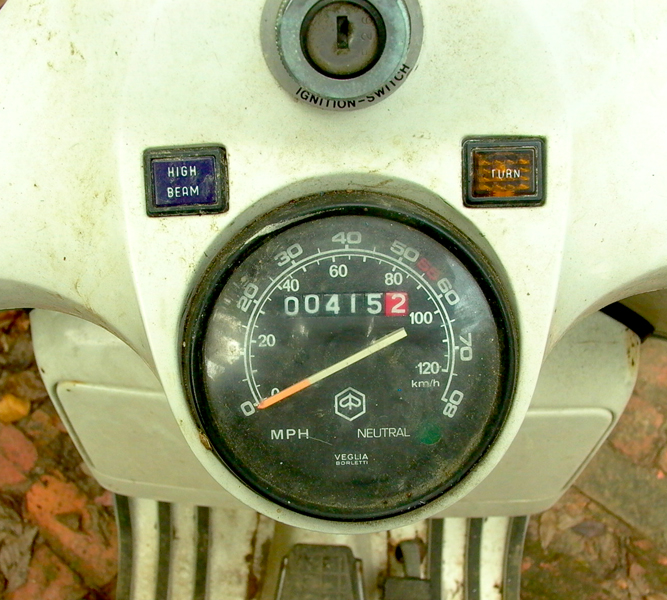In this close-up photograph, a piece of aged industrial equipment takes center stage. The primary focus is a large, circular gauge situated prominently on a grimy, off-white metal surface. Surrounding the gauge, the backdrop features several rusty metal fragments, adding to the equipment's vintage, well-worn appearance.

The gauge, clearly marked with dual measurement systems, ranges from 0 to 80 miles per hour and 0 to approximately 120 kilometers per hour. The lower part of the gauge spells out the word "NEUTRAL," and there’s a distinctive hexagonal symbol with an outlined fly at its center. The brand name "VEGLIA" is displayed at the bottom of the gauge.

Around the gauge, key details include a green square near the 80-mile-per-hour mark and a red number "55" between the 50 and 60 markings. The gauge's mileage reads 4152, indicating its usage history.

Adjacent to this gauge, on the right, is a square button labeled "TURN," and another blue, square button indicating "HIGH BEAM." Above this control panel, a small keyhole is visible, labeled "IGNITION SWITCH," completing the image of a meticulously detailed and storied piece of machinery.